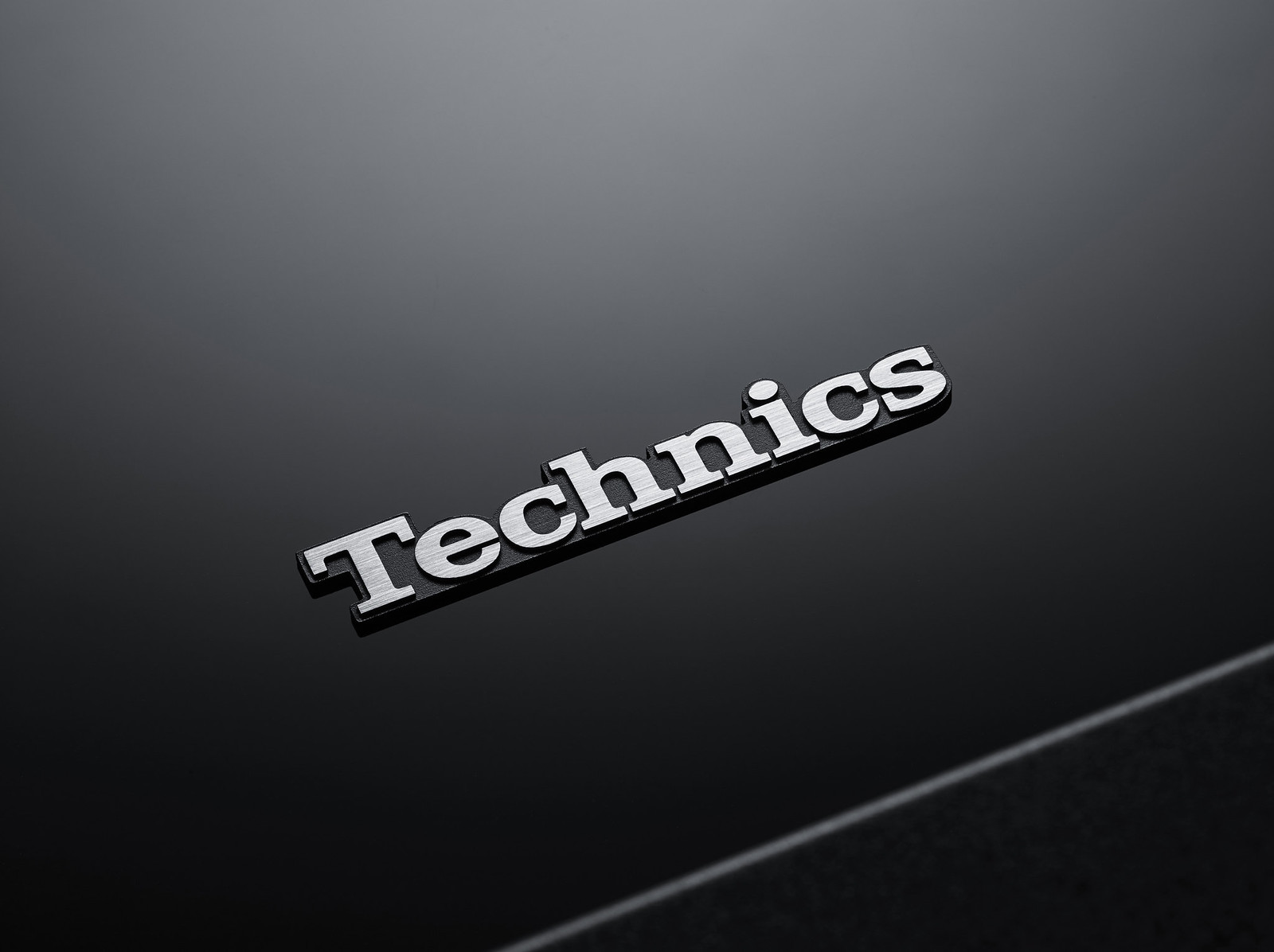The photograph showcases a heavily polished, dark gray metallic surface with the branding "Technics" prominently displayed in the center. The letters T-E-C-H-N-I-C-S, in raised metallic font, each appear to be mounted separately, creating a three-dimensional effect as they slightly pop out from the surface. The brand name is slightly angled, with the "T" positioned towards the bottom left corner and the "S" towards the top right. A diagonal light gray line and a subtle groove run across the bottom right corner of the surface, adding to its sleek, sophisticated appearance. The upper part of the background appears lighter as if illuminated by a diagonal shaft of light, enhancing the visibility of the brand name and adding depth to the image.